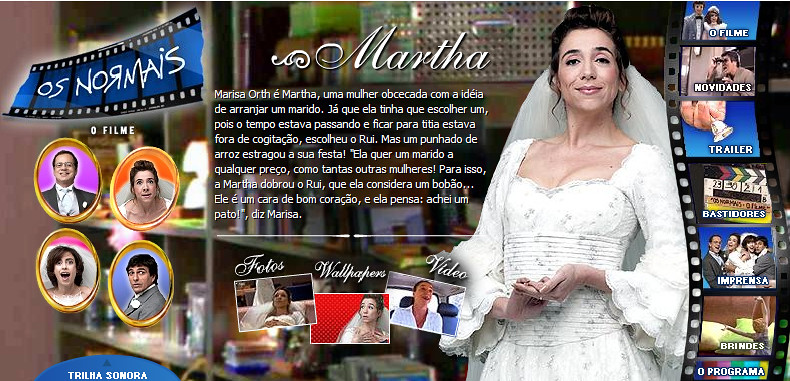A woman stands poised in a form-fitting, white dress that exudes the elegance of a wedding gown, complete with a delicate veil. The dress features a very faint print that adds subtle detail to her sophisticated look. She clasps her hands in front of her and offers a gentle, semi-smiling expression to the camera. The caption identifies her as Martha. 

Surrounding the image is the intricate design of a film strip. On the left side of this film strip, various text elements are displayed: "OS Normase" (with the 'R' rendered backwards), "O-Film," "Crelma Sonora," "Photos," "Wallpaper," and "Video." The right side of the film strip presents additional options: "O-Film," "Movie Duds," "Trailer," "Imprensa," "Brindes," and "O-Programma." 

Centrally placed text, adjacent to the woman in the elegant dress, appears to be in Portuguese, suggesting a Brazilian origin. This combination of motifs and text strongly indicates that the image is an advertisement for "OS Normase."